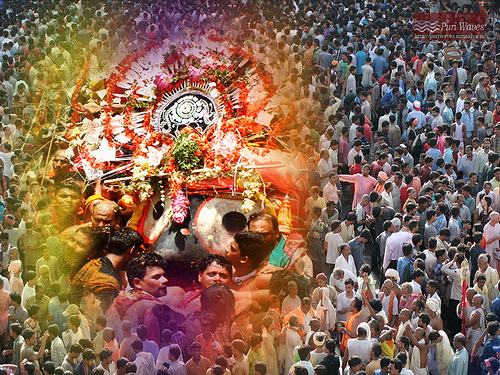The photo captures the vibrant festival of Holi in India, with a large crowd of South Asian men gathered in an open space during the daytime. The crowd appears to be engaged in a significant celebration, possibly a religious ceremony, given the festival context and the worshippers' presence.

Dominating the middle-left section of the image is a superimposed close-up that blends seamlessly into the original scene, creating a composite picture. This overlay focuses on a group of men holding an elaborately decorated object, possibly a statue or a memorial. The object is ornate, featuring black, white, and red colors, adorned with numerous flowers and a decorative headdress. The central motif includes a circle with snake-like structures, surrounded by small rectangular elements and an outer ring with a red dot at the center. Radiating from the circle are metal arcs and red ribbons interwoven with spokes, giving it a dynamic and ceremonial appearance. Below this symbol, there appears to be a drum, emphasizing the rhythmic and celebratory nature of the event.

The photograph also has a transparent overlay on the top right with the text "Pari Waves" in red and white, adding another layer of visual interest to the already intricate and vivid scene.